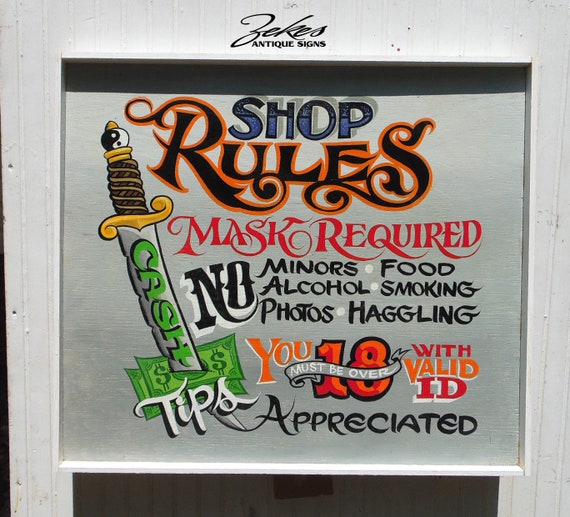The image depicts a square, realistic-looking shop sign with a white wooden background. At the top, the sign reads "Zeke's Antique Signs" in black cursive font. Below this, "Shop Rules" is prominently displayed, with "Shop" in bold blue font and "Rules" in bold black font with orange highlighting. The sign lists several rules in various fonts and colors for emphasis: "Mask Required" in red, "No Minors" in black, "No Food, Alcohol, Smoking, Photos, or Haggling" in different fonts and colors, and "You Must Be 18 with Valid ID" in orange. Towards the bottom, "Tips Appreciated" is written in white font. An artistic illustration of a sword with a yellow handle and a grey blade, featuring a black and white yin-yang symbol, is depicted piercing through dollar bills. The word "Cash" is written in green on the blade. The overall design and typography give the sign a graffiti-like, hand-painted appearance, making it eye-catching but somewhat challenging to read.